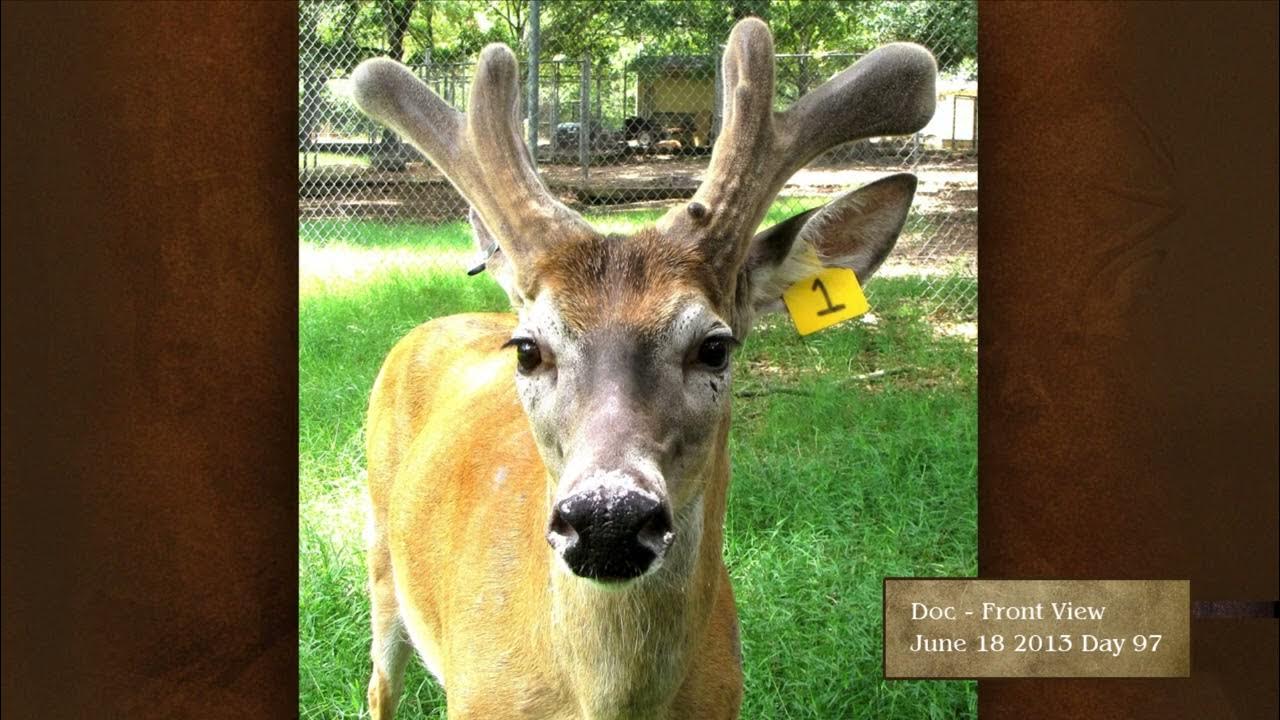The photograph features a young buck deer facing the camera, with its nose close to the lens and slightly turned to the left. The deer, a brown creature with a whitish face and a prominent black nose, sports short, thick, and rounded antlers reminiscent of very thick slingshots on either side of its head. Notably, it has a yellow tag in its left ear, marked with the number "1", that is visible on the right side due to its orientation toward the viewer. The deer stands in a grassy field, characterized by predominantly green grass with some brown patches, and is situated in front of a chain-link fence. Beyond the fence lies a small building with yellow walls and a green roof, surrounded by numerous trees. The photograph is bordered on the left and right by large, brown, leather-like textured rectangles. Additionally, there is a brown rectangle at the bottom right corner inscribed with "dock front view June 18 2013 day 97".